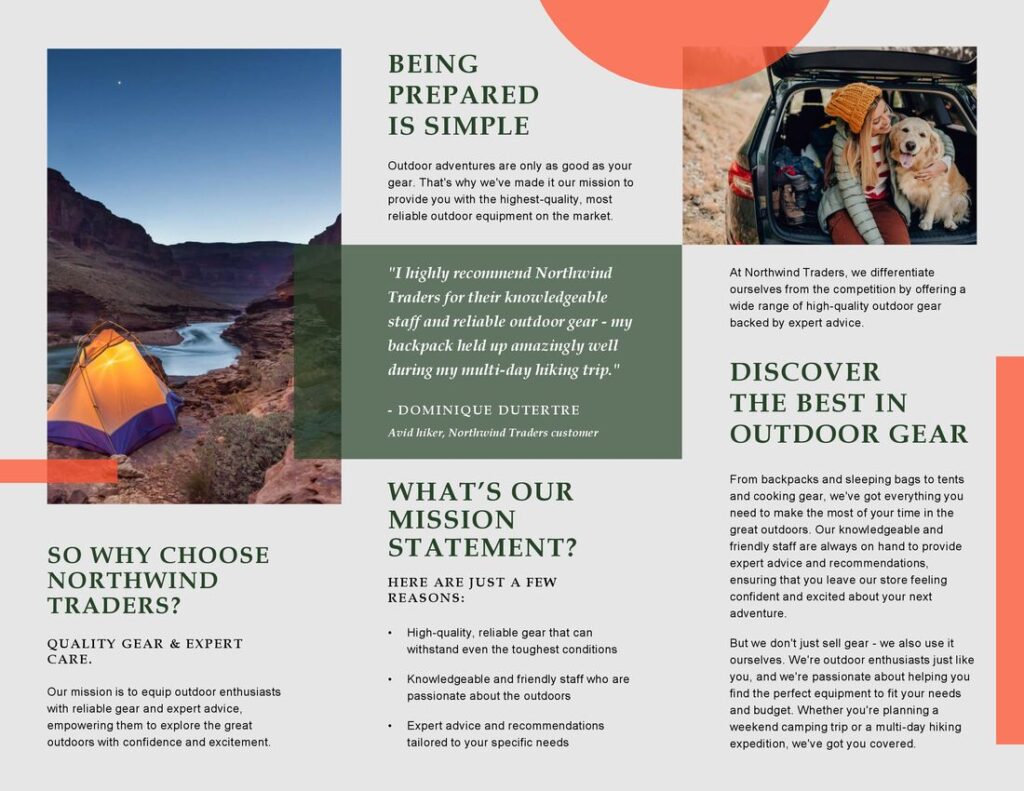In landscape orientation, the image is divided into three distinct columns, creating a card-like layout. The entire background of the image consists of a dark gray hue, seamlessly filling the space from the upper left to the upper right, as well as the lower left to the lower right.

Slightly off-center in the upper portion of the image, an orange half-circle descends, adding a touch of vibrant color. This half-circle is semi-transparent, allowing it to subtly overlay one of the images while still rendering the underlying details visible.

### Left Column:
The left column features an outdoor, camping-themed image extending vertically to the bottom. The scene captures the essence of a serene night in the wild, featuring a light blue, star-studded sky. The middle portion of this column showcases rugged, rocky mountains stretching horizontally, indicative of the challenging yet beautiful terrain. Below the mountains rests a calm water source, reflecting the natural beauty around it. At the bottom left of the image, a tent is pitched, symbolizing a cozy camping spot. Below this picturesque scene, a caption reads:  
"So why choose Northwind Traders? Quality gear and expert care."

### Middle Column:
The middle section of this triptych contains text only, emphasizing the simplicity and mission of the brand. It reads:  
"Being prepared is simple. What's our mission statement?"

### Right Column:
In the upper right-hand corner of the image, a heartwarming scene of a woman and her dog situated in the open hatchback of a car is presented. This captures the spirit of adventure and companionship, accompanied by a caption that invites discovery:  
"Discover the best in outdoor gear."

This richly detailed image offers a compelling blend of visual and textual elements, each contributing to the overall theme of quality and preparedness for outdoor adventures.